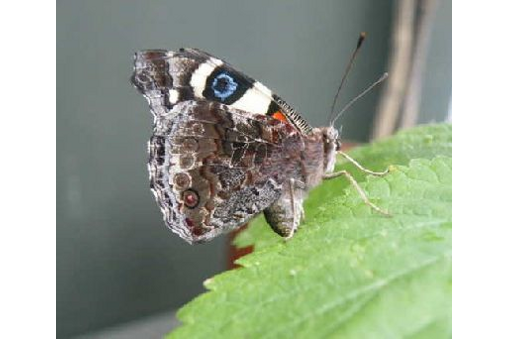This detailed close-up photograph captures a gray-colored butterfly perched delicately on the serrated edge of a green leaf, which occupies the lower right portion of the frame. The background is a smooth gray wall, providing a contrasting backdrop to the butterfly's intricate patterns. The butterfly is facing to the right, with its wings held upright and together, displaying only the upper wing fully. This wing has a camouflaged pattern, primarily gray with hints of brown, along with a noticeable false eye feature. The false eye consists of a black dot surrounded by a light blue ring, encircled by a thicker black ring, and a larger white splotched ring around that. The coloration also includes subtle patches of white, black, and hints of blue and orange near the fringes. The butterfly's body is slightly fuzzy, resembling that of a small bee, with two long antennae that end in bulbous tips sticking out prominently. The front legs are visible, extending outward as it clings to the leaf, making this moment of natural beauty both vivid and captivating.